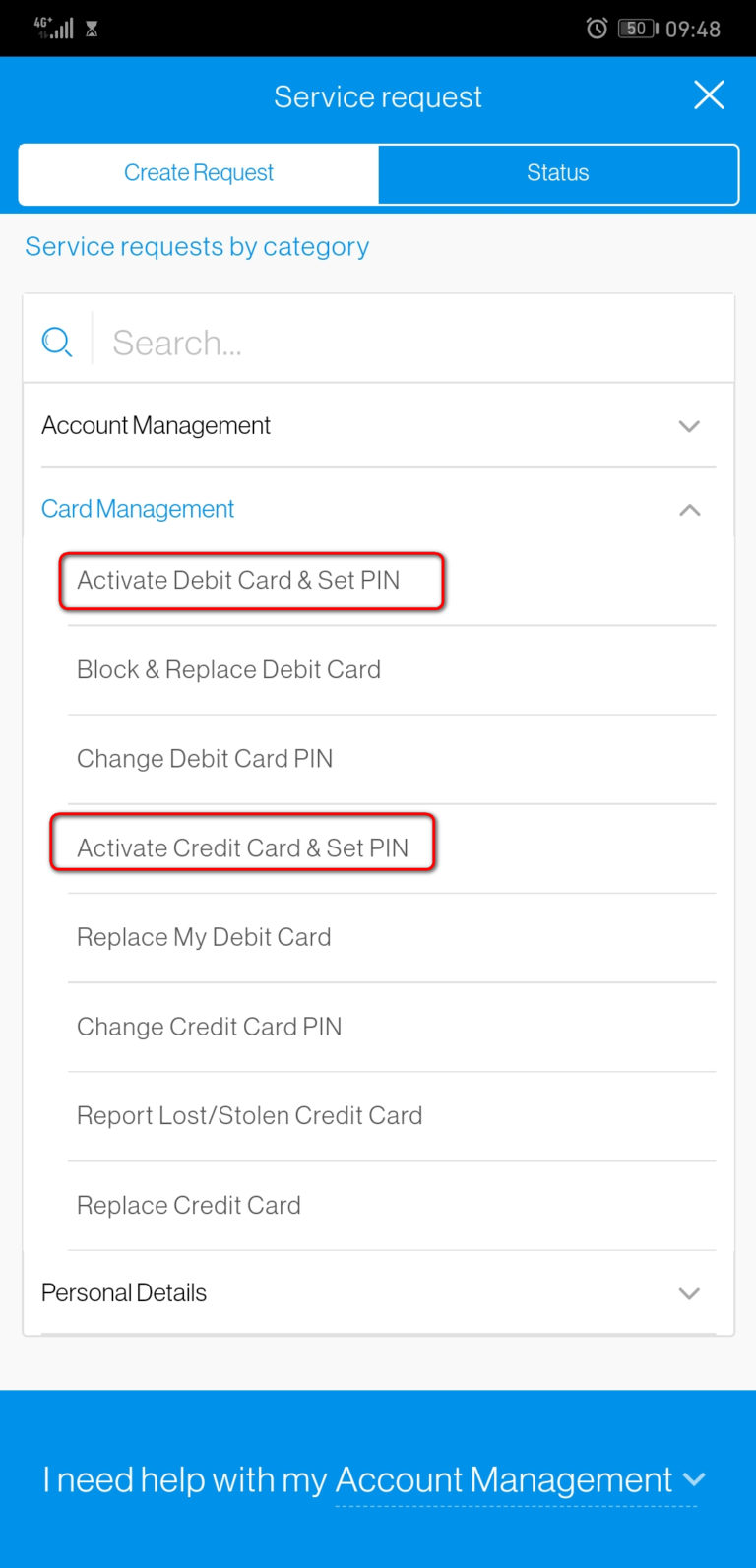This image is a vertically-oriented screenshot taken on a mobile device. At the very top, there’s a thin black bar displaying the time "9:48" on the right-hand side and the signal strength bars on the left. Directly below, a blue rectangle banner with white text reads "Service Request", followed by two options: "Create Request" in white text over a white background, and "Status". 

Below this, a section with a gray background is visible. At the top of this section, in blue text, it says "Service Request by Category", above a menu interface. The menu starts with a search bar, and immediately below are several options listed under "Account Management", followed by "Card Management". Within this section, options are divided into red-encircled categories, the first being "Activate Debit Card and Set PIN".

The options enclosed in the red rectangle under “Card Management” include:
- Block and Replace Debit Card
- Change Debit Card PIN
- Activate Credit Card and Set PIN (also within a red rectangle)
- Replace My Debit Card
- Change Credit Card PIN
- Report Lost/Stolen Credit Card
- Replace Credit Card
- Personal Details

At the bottom of the image, there's a blue rectangle with white text that says, "I need help with my Account Management", notably underlined and with both 'A' and 'M' capitalized.